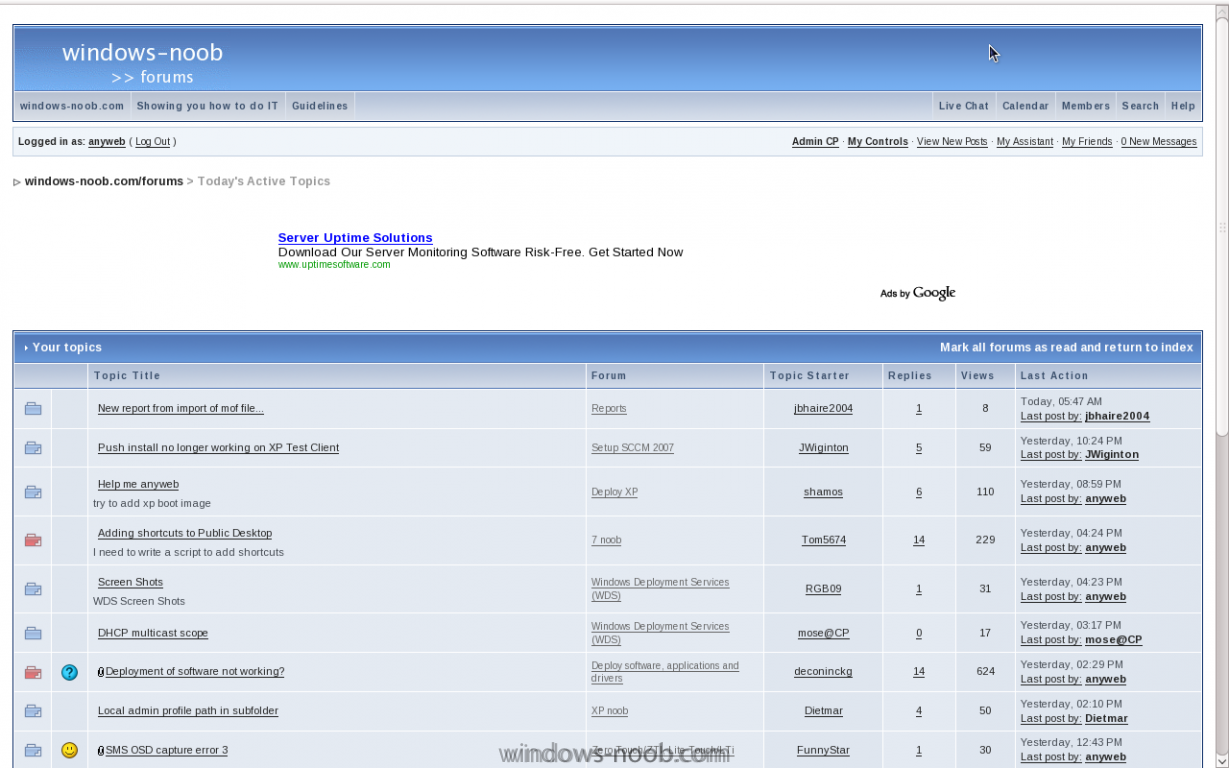A detailed caption for the image could be:

"The horizontal image displays a screenshot of a computer screen showcasing a webpage from Windows-Noob.com. The top section of the webpage features a thin gray line followed by a white background. Below this, there is a prominent blue rectangular horizontal bar. On the left side of this bar, the text 'Windows-Noob' appears in white, followed by '→ Forums' underneath.

Directly below, a darker gray box contains the text 'Windows-Noob.com, sharing how you do it,' and 'Guidelines.' This section is followed by a lighter gray box on the left displaying the text 'Logged in as AnyWeb' in black underlined text, with options to 'click on that' for more details or 'Log out.' Moving further to the right, bold and underlined text options like 'Admin CP' and 'My Control' are visible, alongside other underlined options such as 'View New Posts,' 'My Assistant,' and 'My Friends,' indicating there are zero new messages.

To the left again, 'Windows-Noob.com/forums,' and 'Today's Active Topics' are noted. The middle section prominently features an advertisement with the text 'Ads by Google', followed by a server uptime solutions ad. Below this, a chart with various shades of blue presents a structured layout that includes headers such as 'Your Topics,' 'Link Folders,' 'Topic Titles,' 'Forum,' 'Topic Starter,' 'Replies,' 'Views,' and the 'Last Action.'

The screenshot captures the organized and user-friendly interface of the website, providing a clear view of both navigation options and forum activity details."